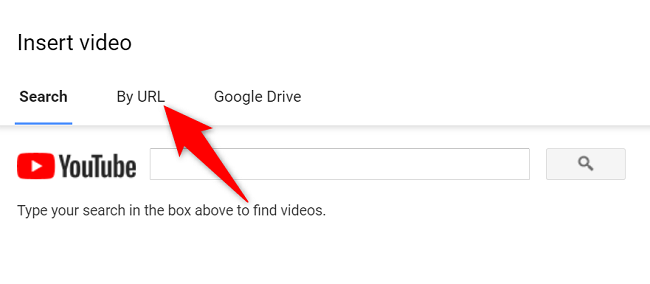A detailed screenshot of a computer interface primarily focused on inserting a video. In the upper left corner, the text "Insert video" appears in black. Below that, there are several distinct sections: "Search" with a blue underline, "By URL," and "Google Drive." A prominent red arrow rises from the bottom center of the image, angled and pointing towards the "By URL" section, indicating the option to use a URL for video insertion. In the left-center of the image, a red square with a white triangle in the middle represents the YouTube logo. To its right, the word "YouTube" is displayed in bold black capital letters. Dominating the center is a large search box with an adjacent magnifying glass icon. Beneath this search box, the instruction "Type your search in the box above to find videos" is visible. The red arrow is long, narrow, and points directly to "By URL" at its wide top, providing guidance on finding videos through a URL input.